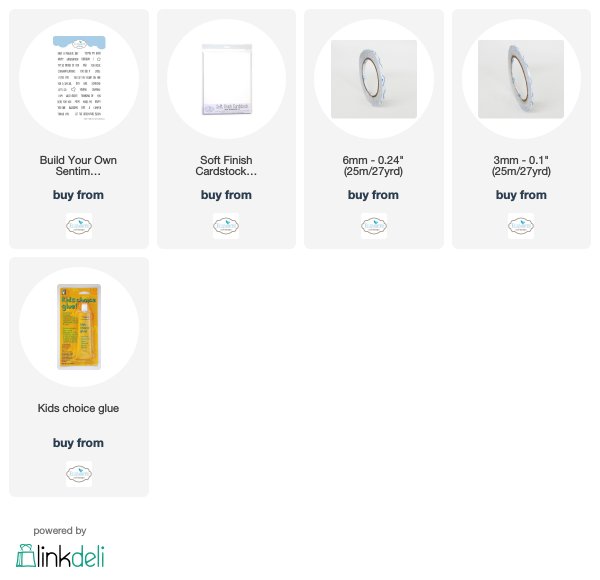The image features a white background with two rows of vertically aligned rectangular items. The top row includes four items, and the bottom row contains one. Each item is gray with a circle at the top. Below the circle, there's black font detailing the product, followed by a “buy from” link and a logo, which is consistent across all items.

1. **First Item (Top Left)**:
   - **Header**: "Build Your Own S-E-N-T-I-M..."
   - **Content Within Circle**: Unclear, but includes black font and a blue header.
   - **Link Below**: "Buy from" with the repeated logo.

2. **Second Item (Top Second)**:
   - **Header**: "Soft Finish Card Stock..."
   - **Appearance**: Resembles a tablet.
   - **Link Below**: "Buy from" with the same logo.

3. **Third Item (Top Third)**:
   - **Header**: "3 millimeter - 0.24 inches (25M/27 yards)"
   - **Appearance**: Roll of tape.
   - **Link Below**: "Buy from" with the consistent logo.

4. **Fourth Item (Top Fourth)**:
   - **Header**: "33 millimeter - 0.1 inches (25 millimeter/27 yards)"
   - **Appearance**: Another roll of tape with different dimensions.
   - **Link Below**: "Buy from" with the same logo.

5. **Fifth Item (Bottom)**:
   - **Header**: "Kids Choice Glue"
   - **Link Below**: "Buy from" with the consistent logo.

In the bottom-left corner of the image, there is a logo indicating "Powered by LinkDeli" which features a green shopping bag, with the word "deli" in green.